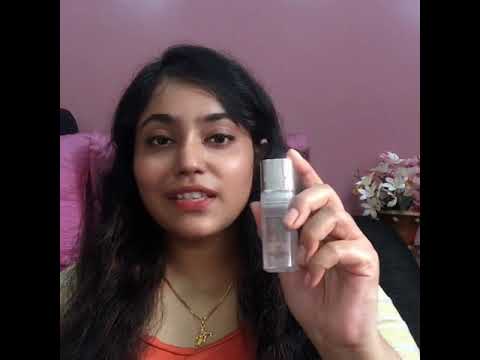The photograph captures the upper body of a young woman seated against a pink and lavender-toned background. She is centered in the image, showcasing a clear bottle with a white cap, which appears to be a beauty product or perfume, in her right hand. The woman, who has lightly tanned white skin and long black wavy hair tucked behind her ears, is adorned with a gold pendant necklace. She wears an orange tank top with a v-neckline. Behind her, a rear wall is decorated with pink wallpaper, and to the right, a vase with white and pink flowers adds a delicate touch. The scene appears to be set indoors and gives the impression of a casual vlog or product review setup.